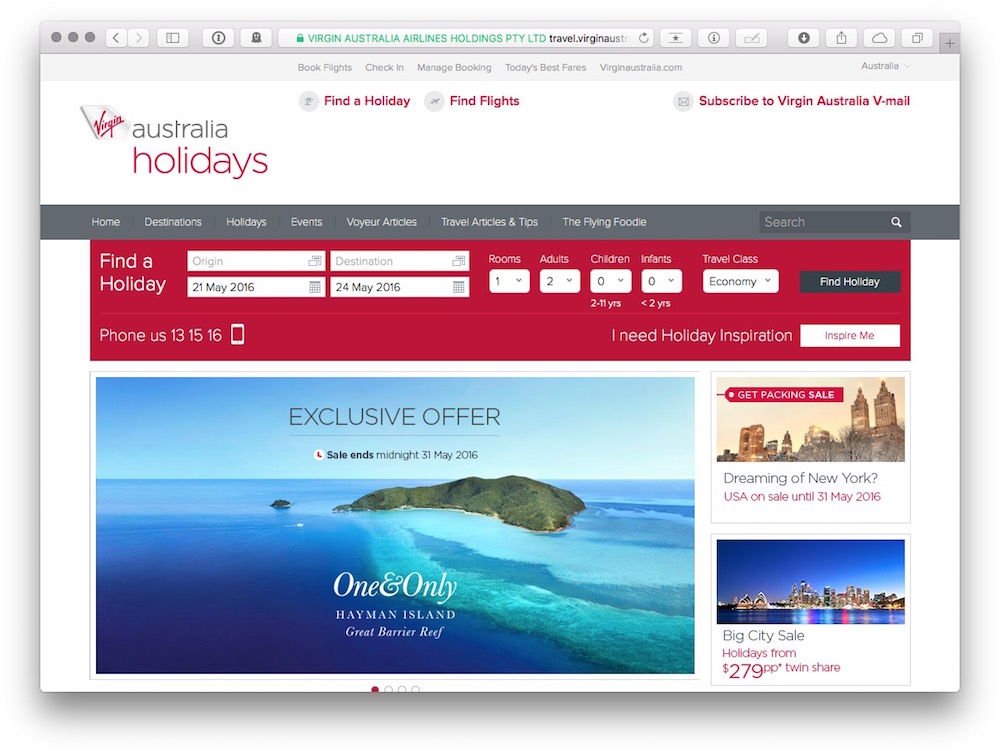The image is a detailed layout featuring various elements associated with the Virgin Australia brand. Towards the left, the prominent Virgin Australia logo is displayed on a slanted white background. The logo features the word "Virgin" in red, italicized font with the right side of the 'V' elongated over the rest of the letters. Below this, "Australia" is written in a smaller, grey font. Beneath "Australia," the word "holidays" appears in larger, bold red text.

To the right of the logo, there's a text that reads "Find a Holiday" in bold red font accompanied by a light grey circular icon with a palm tree. Further right, the text "Find Flights" is similarly bold and red, paired with a light grey circular icon depicting an airplane. Moving rightward still, the phrase "Subscribe to Virgin Australia V-Mail" is displayed in bold red font, flanked to its left by a light grey circular icon showing an envelope.

Below these sections, a medium grey heading features multiple white text menu options: from the left, the options include Home, Destinations, Holidays, Events, Voyeur Articles, Travel Articles and Tips, and The Flying Foodie. On the far right of this menu is a search query option with a light grey box and the word "Search" in lighter grey, accompanied by a white magnifying glass icon.

The next section transitions into a functional search area for flights. It prominently displays "Find a Holiday" in white font against a red background. A dark grey circular icon on the far right reads "Find Holiday" in white text. Towards the bottom of this section is a call-to-action button with the phrase "I Need Holiday Inspiration" in white, flanked by a white icon containing red font that says "Inspire Me". The overall background of this area is dark grey, creating a cohesive and visually striking design.

This comprehensive layout effectively guides users through various features and services offered by Virgin Australia, combining visual elements and text to create an engaging and user-friendly interface.